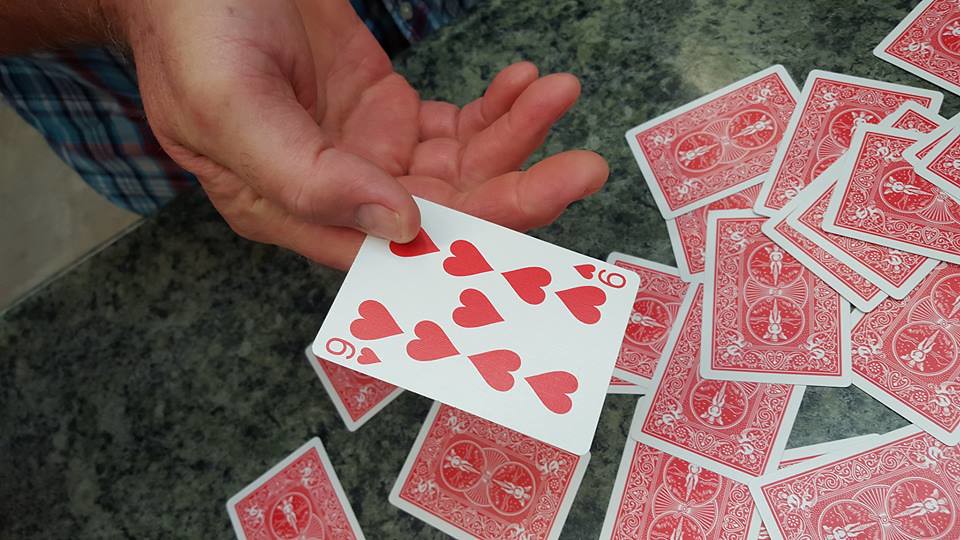The image depicts a person seated at a marbled granite table, strewn with a deck of black and white cards laid face down. In their hand, they prominently display the Nine of Hearts, the sole card facing upwards. The individual's fair-skinned hand contrasts with the sleek, granite surface. The person's attire is partially visible, showcasing a predominantly blue, multicolored flannel shirt. The focal point of the image is the Nine of Hearts, centrally positioned and sharply in focus, while the surrounding face-down cards create a scattered, textured background on the elegant counter.